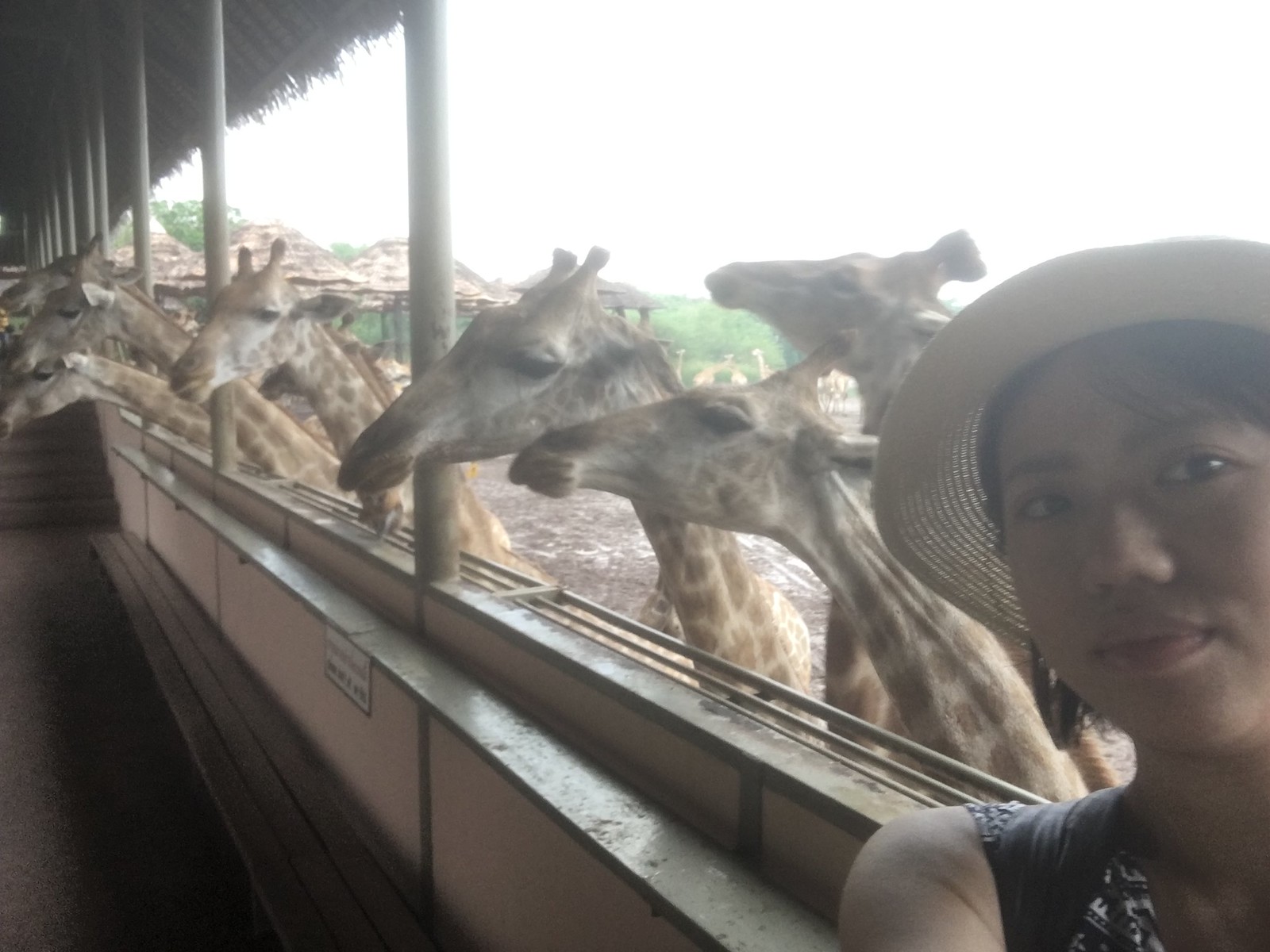In this photograph, an Asian woman takes a selfie in the bottom right corner, capturing her smiling face adorned with a beige-brimmed hat and a sleeveless black tank top. Her brown hair peeks out from under the hat as she stands near a zoo enclosure. Behind her, seven giraffes with yellow fur and brown spots lean over a gray partition wall with pink accents. These giraffes, characterized by their black eyes and short, stubby horns, appear curious and eager, seemingly reaching out to be fed. The backdrop includes a grass-thatched awning supported by beige poles, and the environment features a brown, muddy ground with additional bamboo-roofed shelters and green foliage. The sky above is a clear white, completing the vibrant scene.